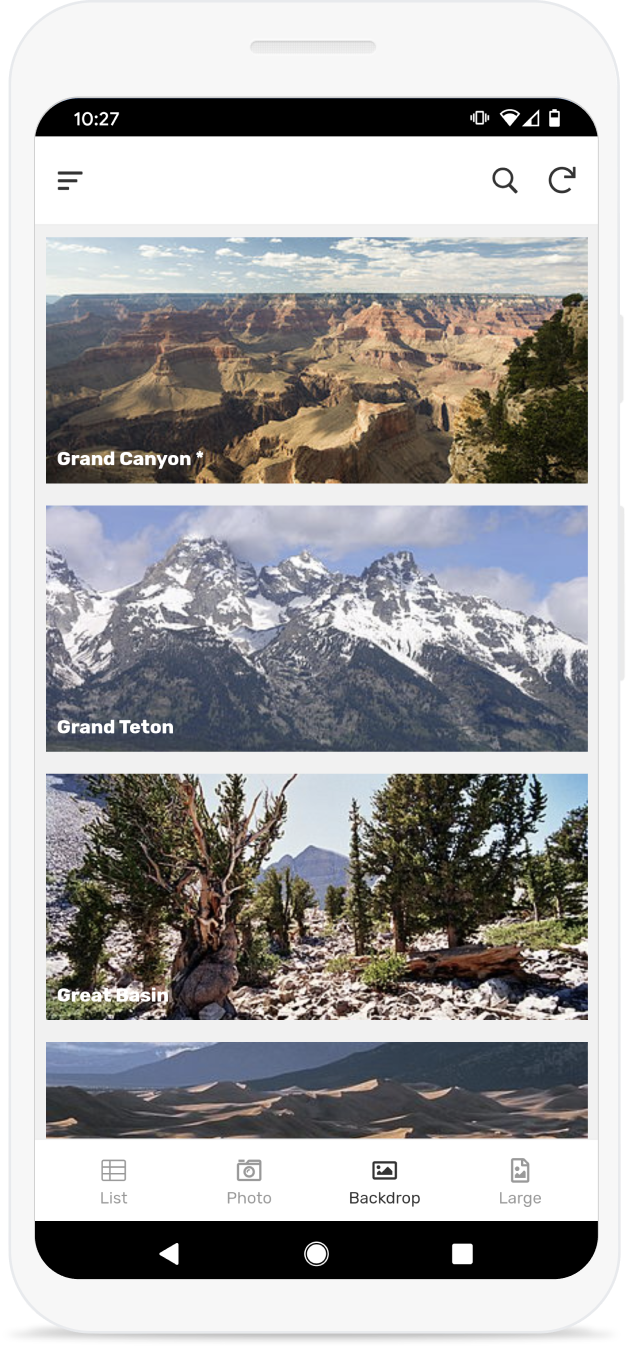The image depicts a smartphone screen with the time displayed as 10:27 in the upper left-hand corner. The screen showcases a webpage or an app interface characterized by a primarily white background, featuring white banners at the top and bottom of the page. 

The main content area displays three full photographs and one partial photograph at the bottom. The top photograph is an iconic view of the Grand Canyon, labeled "Grand Canyon" in the lower left-hand corner. Following below is a stunning picture of the Grand Teton, similarly labeled "Grand Teton." The third photograph shows the rugged beauty of the Great Basin, with the label "Great Basin." The partially visible photograph at the bottom hints at a desert landscape.

Prominently, there are four icons positioned below the photographs, labeled "List," "Photo," "Backdrop," and "Large." The "Backdrop" icon is highlighted, indicating it is the currently selected option.